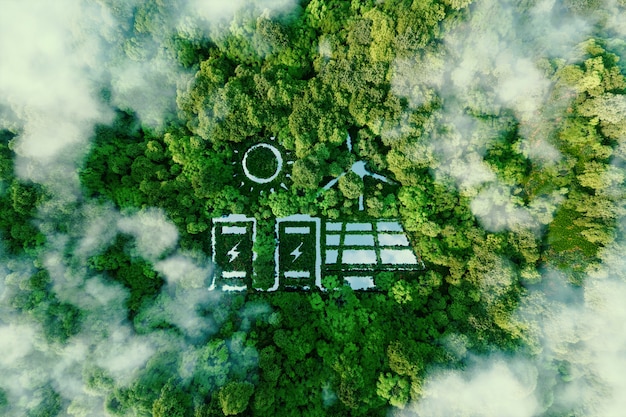This image is an aerial, photorealistic illustration of a dense forest, capturing a vibrant gradient of greens from deep to light shades. The forest canopy is enveloped by clouds resembling steam rising off the trees, enhancing the ethereal atmosphere. At the center, partially obscured by the dense foliage, are multiple objects suggestive of renewable energy sources: two shapes resembling batteries, an array of solar panels, what appears to be a wind turbine, and a round spiked object reminiscent of the sun. This clustered assembly evokes an unfinished or abandoned effort to construct something. The bright green, white, and black color palette emphasizes the contrast between the natural environment and these artificial structures, likely symbolizing a promotional message advocating for clean energy.